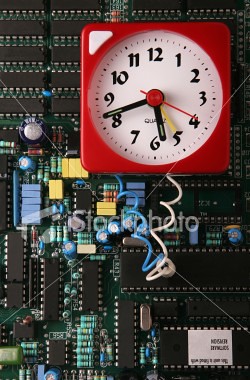The image features a complex mechanical setup resembling a circuit board or the inner workings of a sophisticated machine dominated by various interconnecting colorful parts, including dots, lines, and gear-like components in yellow, blue, green, and gray shades. Prominently, there is a square clock with a red exterior frame and a white circular face situated at the upper right side. The clock displays black numbers and hands, save for a red second hand. Additionally, distinguishable wires, one turquoise and one white, emerge from the clock, integrating with the surrounding mechanical elements. Notably, in the lower right-hand corner, there is a small white area with lettering, adding to the detailed intricacies of the setup.